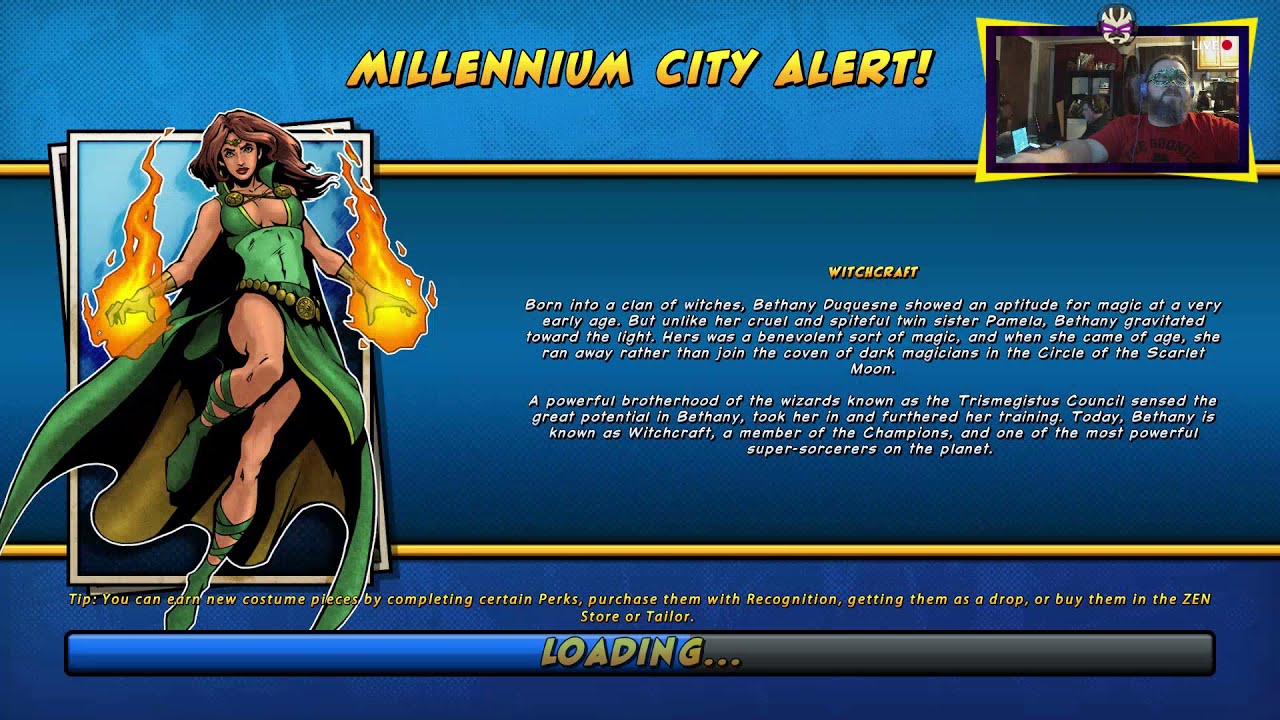The image is a screenshot from a video game, featuring a "Millennium City Alert" notification at the top in bold yellow cartoon font with an exclamation point. Below this header, there's an extensive explanation labeled "Witchcraft," detailing the character Bethany Duquesne’s backstory as a benevolent witch who fled her dark coven to join the Tri-Megistus Council and becoming one of the most powerful super-sorcerers as part of the Champions. Dominating the left side of the screen is an illustrated character card against a blue background, showing Bethany mid-air with long brown hair, a green cape, and a superhero uniform, emitting flames from her outstretched hands. On the upper right, there's a small rectangular box displaying a live stream with a man in a red t-shirt, sporting a beard, glasses, and headphones, presumably playing the game from his home setup. At the bottom of the image, a loading bar progresses with the word "Loading..." in yellow, and beneath it, there's a tip about earning costume pieces in the game. The overall scene suggests an engaging, detailed RPG or superhero-themed game with real-time elements and rich character lore.